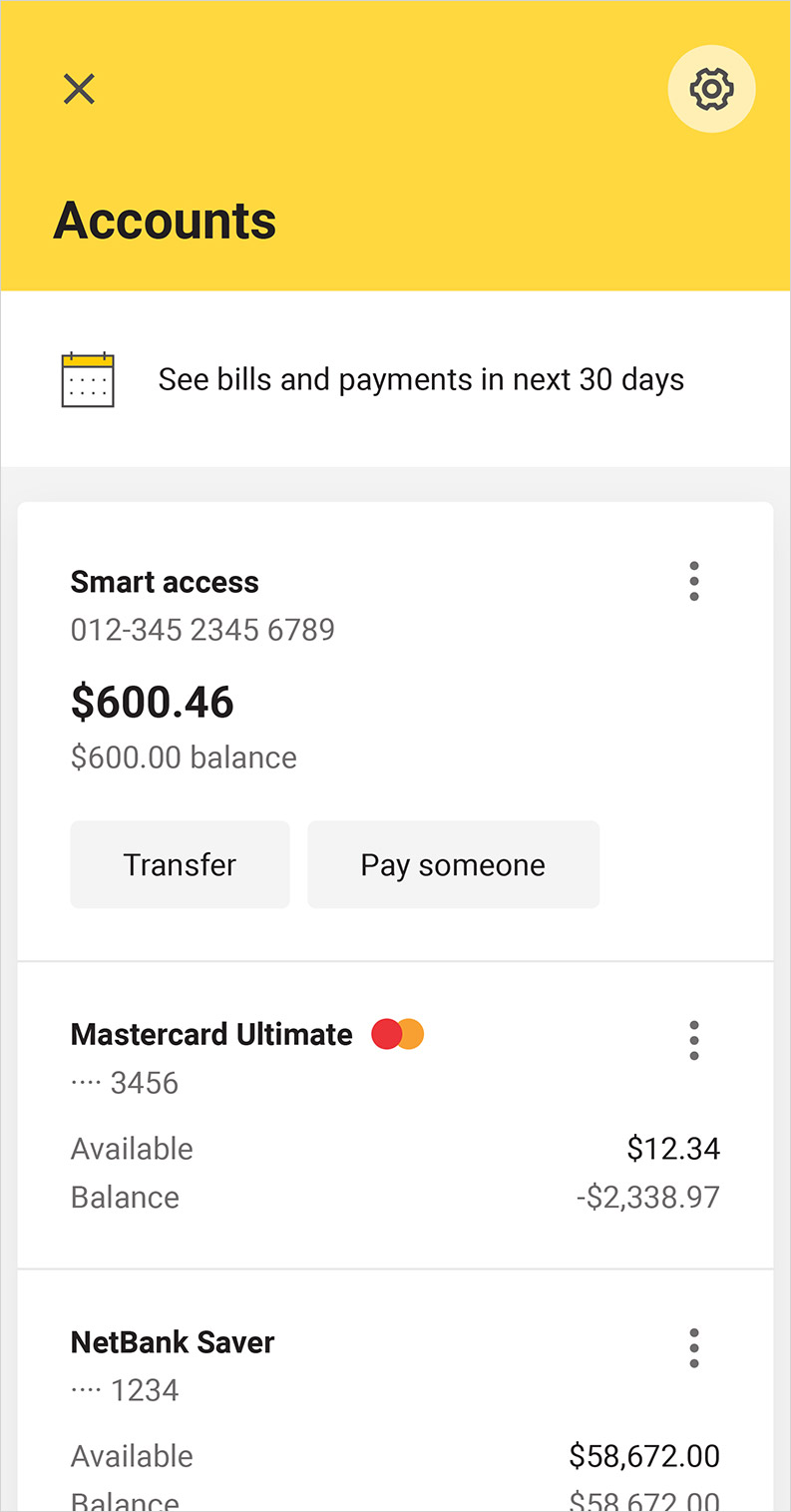The image is a vertically oriented screenshot from a mobile phone displaying the "Accounts" tab. The header is yellow, featuring an 'X' close button in the upper left corner and a settings button in the upper right. Centered below the header, in bold black font, is the word "Accounts." A white background extends below with text that reads "See bills and payments in next 30 days," accompanied by a calendar icon to the left.

Below this section, three accounts are listed within separate white boxes:

1. **Smart Access**: 
   - **Balance**: $600.46 
   - **Options**: 'Transfer' button, 'Pay Someone' button 
   - **Additional Feature**: Three vertical dots in the top right corner of this section for more options.

2. **MasterCard Ultimate**: 
   - **Logo**: MasterCard logo with red and yellow circles on the right side.
   - **Card Number**: Last four digits - 3456
   - **Available Balance**: $12.34 
   - **Current Balance**: -$2,338.97 

3. **NetBank Saver**: 
   - **Available Balance**: $58,672.00 
   - **Current Balance**: $58,672.00

The entire bottom section is outlined with a thin gray border, clearly demarcating the end of the accounts list.